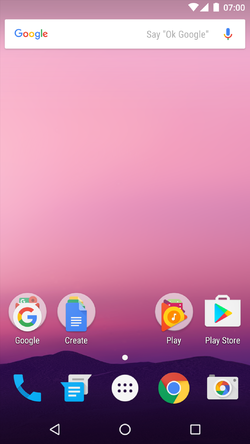A high-resolution screenshot of a smartphone's home screen, likely an Android device, showcases a serene background image of a silhouetted mountain range in dark purple hues. The sky above the mountains is a lighter shade of purple, creating a tranquil gradient effect.

At the very top of the screen, a white Google search bar is prominently displayed, featuring the text "Say 'OK Google'" and a microphone icon for voice searches. Above this search bar, the smartphone's status icons are visible, including the time, which reads "07:00," and indicators for battery life, Wi-Fi connectivity, and other standard notifications.

The home screen is minimalistic, with only a few app icons neatly arranged. On the top row, there is the colorful Google app icon and a Google Docs icon labeled “Create.” Below these, the Play Store icon is prominently featured. At the bottom of the screen are four essential icons: a phone icon for making calls, a camera icon, and another instance of the Google app icon. The sparsely populated home screen exudes a clean and organized aesthetic, emphasizing functionality with essential apps easily accessible.